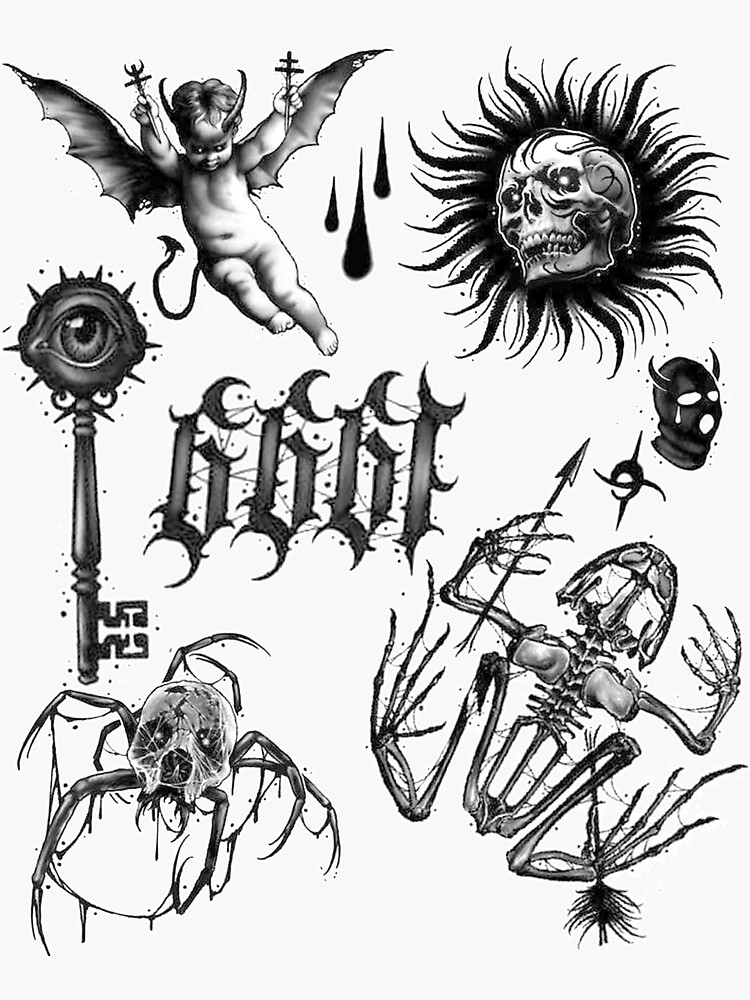The composite image features an eclectic assortment of intricate drawings scattered sporadically across the canvas. Dominating the upper left section is a whimsically sinister baby devil, complete with bat-like wings, curled horns, a forked tail, and clutching two objects reminiscent of twisted crosses. In the top right corner, a menacing skull is encapsulated within a razor-sharp circular design, emanating an aura of danger. Further adding to the macabre collection, a skeletal frog and a spider's exoskeleton contribute to the eerie theme. Additionally, there is a surrealistic key, with an eye seamlessly integrated into the bow – the part meant for gripping – imbuing the otherwise ordinary object with an unsettling, lifelike quality.